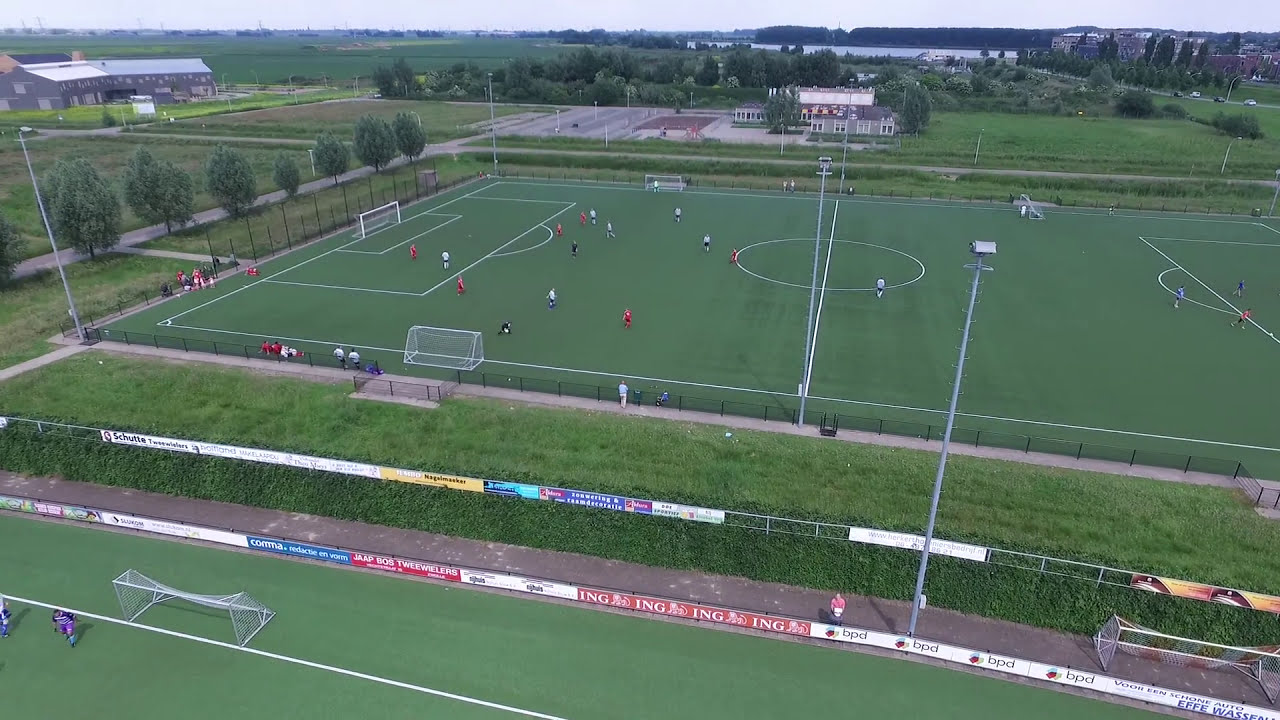The aerial photo captures a vivid scene of two adjacent soccer fields, emphasized by their striking green artificial turf and crisp white chalk outlines. The viewer's perspective, likely from a drone, offers an expansive view, though the left field is partially cropped, revealing only a sliver of green and a goalpost with two individuals nearby.

The main focus is on the uncropped right field, teeming with the energy of a soccer match. Players in red and white jerseys dominate the scene, with additional figures in black, possibly referees, adding to the dynamic palette of colors. The players congregate mainly towards the center left of the field, where the action seems concentrated. On the sidelines, a few onlookers can be spotted, adding to the liveliness of the scene.

In the distant background, a series of landmarks enrich the photo. To the top center and left, a large white building is flanked by a sprawling parking lot. To the far left, a gray, two-story building with a white roof stands tall. The backdrop also hints at a serene landscape with farm-like fields, a meandering road, and a discernible lake at the very top center. The skyline stretches across the image, enshrouded in a blanket of clouds, lending a muted, grayish tone to the otherwise vibrant photograph.